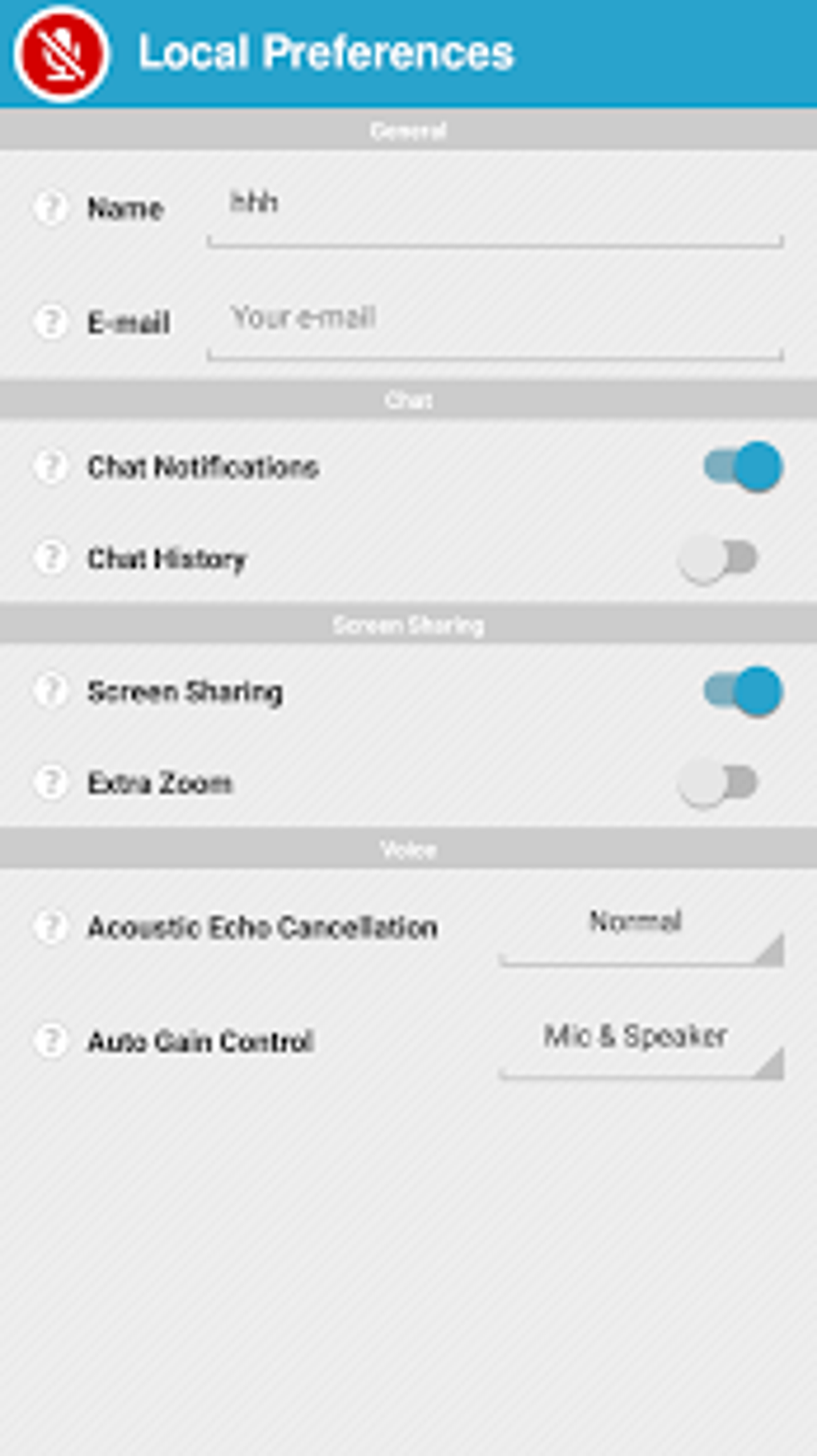The image depicts a user interface screen designed for adjusting local preferences, featuring a blue header with the title "Local Preferences" written in white at the top center. 

On the right side of the header, there's a red circle outlined in white, containing a white microphone icon with a strike-through, indicating that the microphone is turned off.

Below the header, there is a form with various settings:

1. **Name:** Listed as "BHH".
2. **Email:** A field for entering an email address.
3. **Chat Notifications:** A toggle switch set to "On," displayed in blue.
4. **Chat History:** A toggle switch set to "Off," displayed in grey.
5. **Screen Sharing:** A toggle switch set to "On".
6. **Extra Zoom:** A toggle switch set to "Off".

At the bottom of the form, there are further settings:

- **Acoustic Echo Cancellation:** Set to "Normal".
- **Housekeeping Control:**
  - **Mic and Speaker:** These are split into two sections - "General" and "Voice".
    - Under **General**:
      - **Name and Email:**
      - **Chat:**
        - **Chat Information:** Includes toggles mentioned above.
    - Under **Voice**:
      - **Sound Recording:**
      - **Extra Screen Sharing:**
      - **Echo Cancellation:**

The interface ensures the user has comprehensive control over chat and voice-related settings, providing a clear and organized layout for easy adjustments.